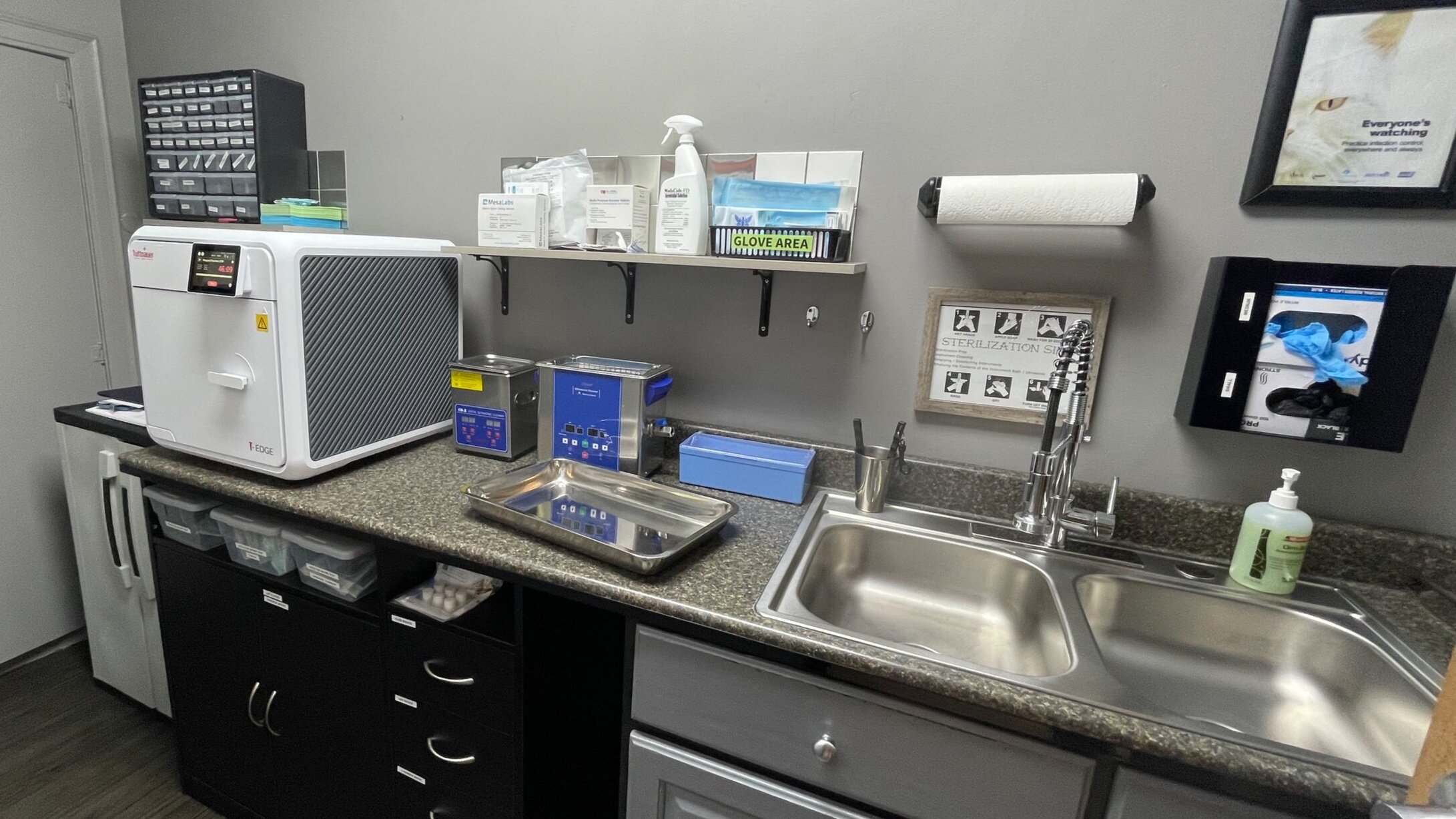The image depicts a meticulously organized medical or veterinary office, featuring a sterilization station centered around a large industrial steel sink. Above the sink, there's a roll of paper towels and a sign outlining best practices for hand washing. To the left, a poster with a white cat in a black frame humorously titled "Everyone's Washing" is prominently displayed. The countertop, possibly granite, is accompanied by a metal tray with what appears to be a sharps container, a spray bottle, and several labels detailing the "glove area" which includes boxes of blue reusable gloves. Additionally, various blue and steel equipment is strategically placed, indicating potential uses for different medical procedures. Below the countertop, a series of black drawers, neatly labeled, house small tubs containing essential items. The entire setup conveys a very clean, sterile, and orderly environment, suggesting active preparation or ongoing processes within the office. A white doorway and wall are visible in the background, contributing to the overall crisp and clinical atmosphere.